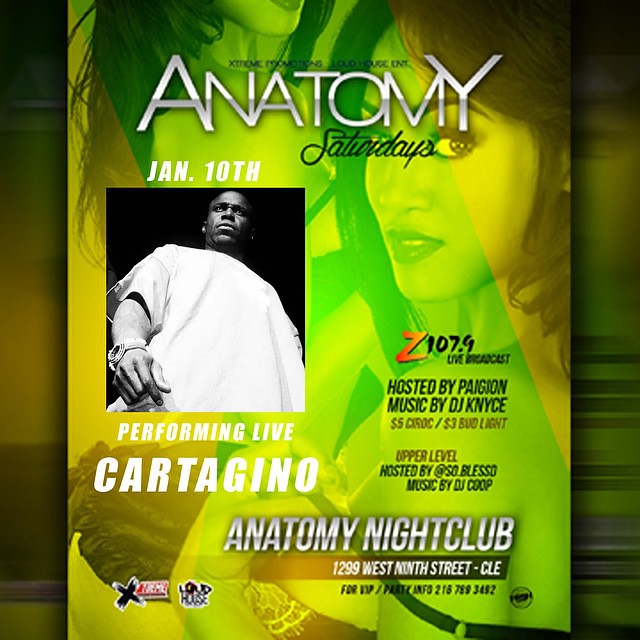The poster is an advertisement for the Anatomy Nightclub's event on Saturdays, specifically January 10th, featuring a live performance by Carte de Genome. The design of the poster is primarily in shades of yellow and green, with detailed overpainted images of scantily clad women in black lingerie superimposed in the background. Dominating the top half of the poster is a photograph of a serious-looking, seemingly bald African-American gentleman in a white t-shirt and a large watch on his right wrist. To the right of his image, the text mentions Z-107.9 and that the event is hosted by Pagan Music, featuring DJ Nice, with drink specials listed as $5.00 Cirque and $3.00 Bud Light. The upper level is hosted by SL Russo with music by D-Stop. Finally, the nightclub's location is clearly stated as Anatomy Nightclub, 1299 West 9th Street, Cleveland.